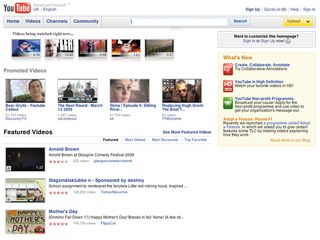Screenshot of a YouTube User Interface: 

The image displays a YouTube interface featuring several key sections, though the text and images are somewhat blurry and hard to read. At the top, the YouTube logo is visible with the letter 'U' in black and a white box containing 'tube,' followed by text suggesting the region as 'UK' with a faint vertical line that reads 'English.' Next to this logo, there are buttons for 'Sign Up' and 'Sign In.'

On the left, there are five small, indistinct thumbnails under a section labeled 'Videos Being Watched Right Now.' Below this, there is another section titled 'Previously Viewed Videos' with four thumbnails. Further down, there’s a section named 'Featured Videos,' displaying three videos each marked with different star ratings.

On the far right, there's a 'What's New' box featuring three small icons accompanied by some unreadable text. 

At the top of the interface, there are navigation buttons for 'Home,' 'Videos,' 'Channels,' and 'Community,' all represented by gray buttons with blue text. Additionally, there is a white search box with a blue search button and a yellow upload box that appears to have a dropdown menu.

Overall, the entire interface is challenging to read due to the small, blurry text and indistinct images.